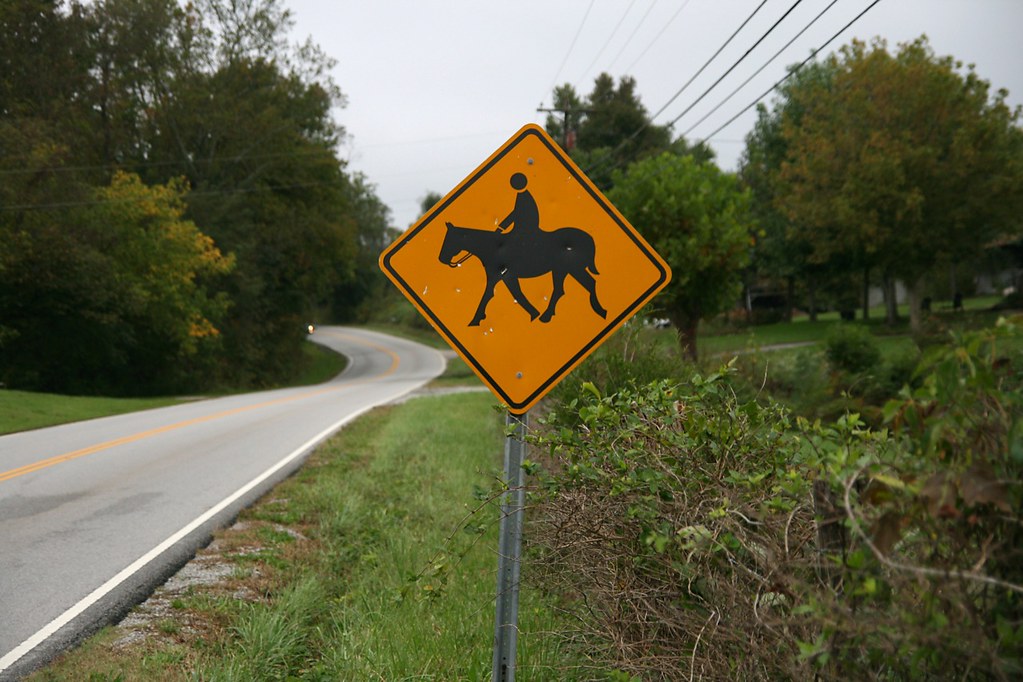This horizontally rectangular exterior image captures a serene scene under natural lighting with an overcast sky. From the lower left of the image, a two-lane road with a prominent double yellow line extends towards the center before curving gently back to the left. To the right of the road, there is a grassy shoulder area, which transitions further right into dense shrubbery and several large, lush green trees in the background. In the foreground, at the center of the frame, stands the upper portion of a metal street signpost. Affixed to the top of the post is a distinctive square yellow sign, oriented so that its corners point upward and downward. The sign features a black border and depicts an image of a man riding a horse, with both the rider and the horse facing the left side of the frame.